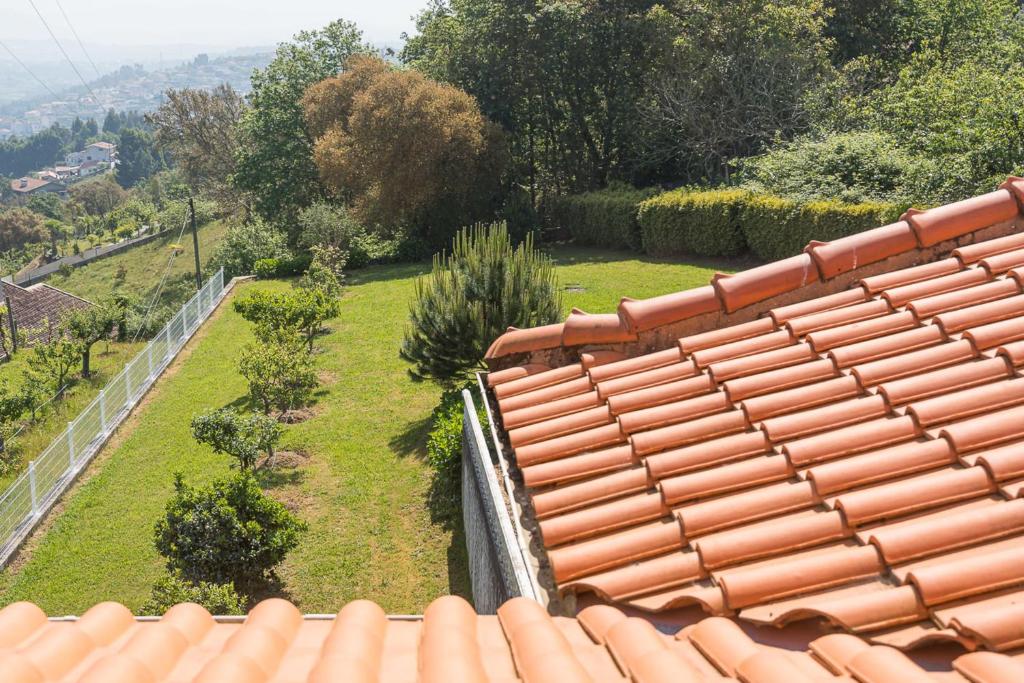The photograph, taken during daylight from the roof of a house or structure with terracotta clay tiles resembling those common in Spain, captures a well-maintained, fenced-in yard. The roof slopes down, offering an angle that reveals a lush green lawn, meticulously mowed and surrounded by a white fence partially covered by carefully trimmed hedges. Within the yard, several saplings and small trees of various shades of green are visible, some bluish-green and others yellow-green or even brownish. 

On the right side of the yard, a hedge line borders the property, leading to a dense wooded area. To the left, a low fence doubles as a retaining wall before it drops off into another person's yard below, also lined with young trees. From this elevated vantage, one can see into a valley that stretches out to reveal more trees, shrubs, and distant buildings hard to distinguish due to their distance. The valley's far end shows a misty or smoggy landscape, culminating in what appears to be mountains in the backdrop under a bright, sunny, grayish-blue sky. There are no people or animals present, and the photograph boasts excellent lighting and focus, enhancing the tranquil beauty of the scene.